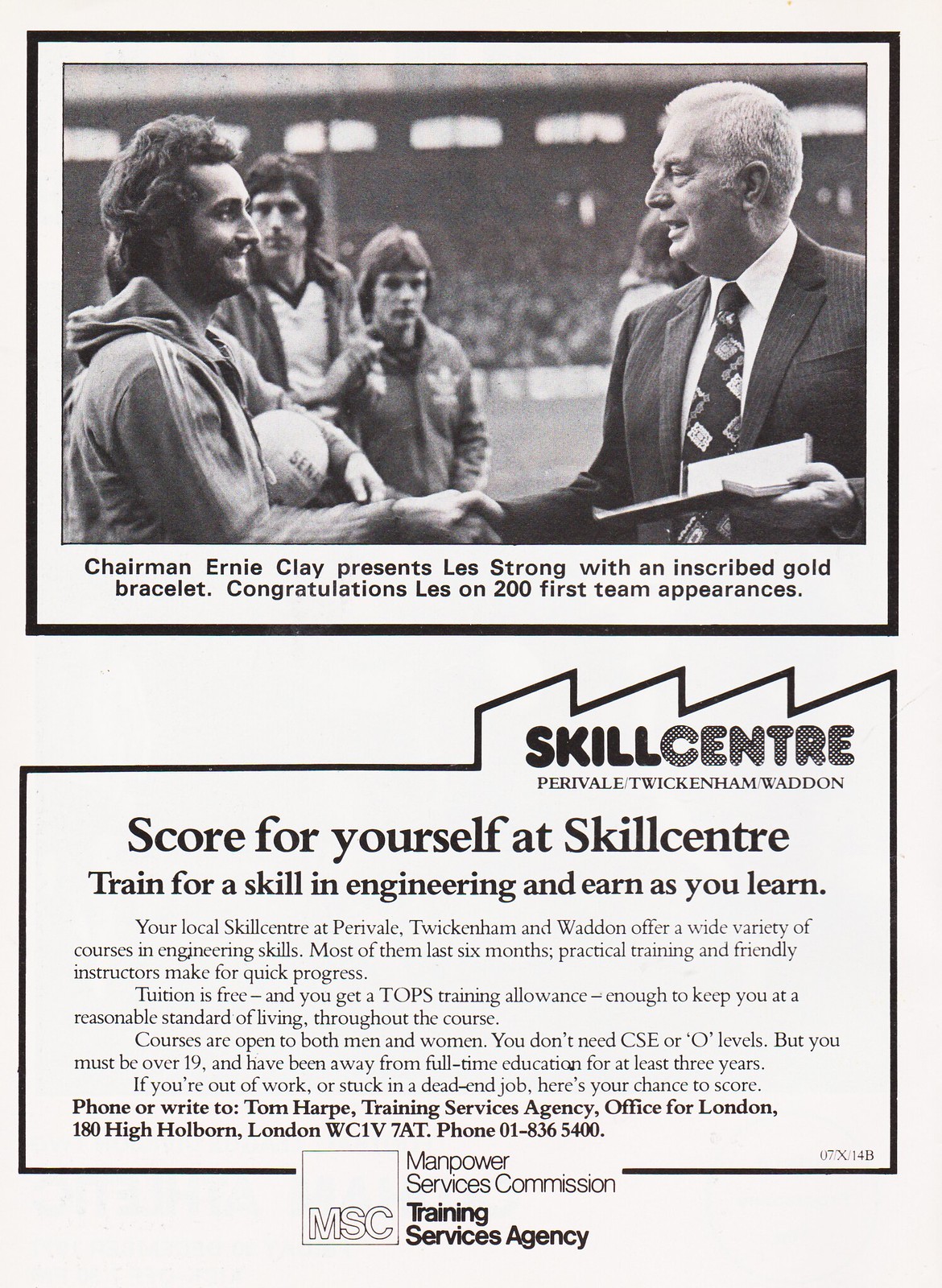This black-and-white image appears to be a page from a magazine, pamphlet, or program from the late 1980s or early 1990s, notable for its vintage aesthetic. At the bottom, there's an advertisement for the Skill Center, offering training services. The ad features a photograph of Chairman Ernie Clay presenting Les Strong with a gold bracelet, suggesting some form of achievement or recognition. The design, fonts, and overall style are reminiscent of publications from the 1990s. The content, including an address and phone number, indicates that this material originated in London, further emphasized by its distinctly non-American format and layout.